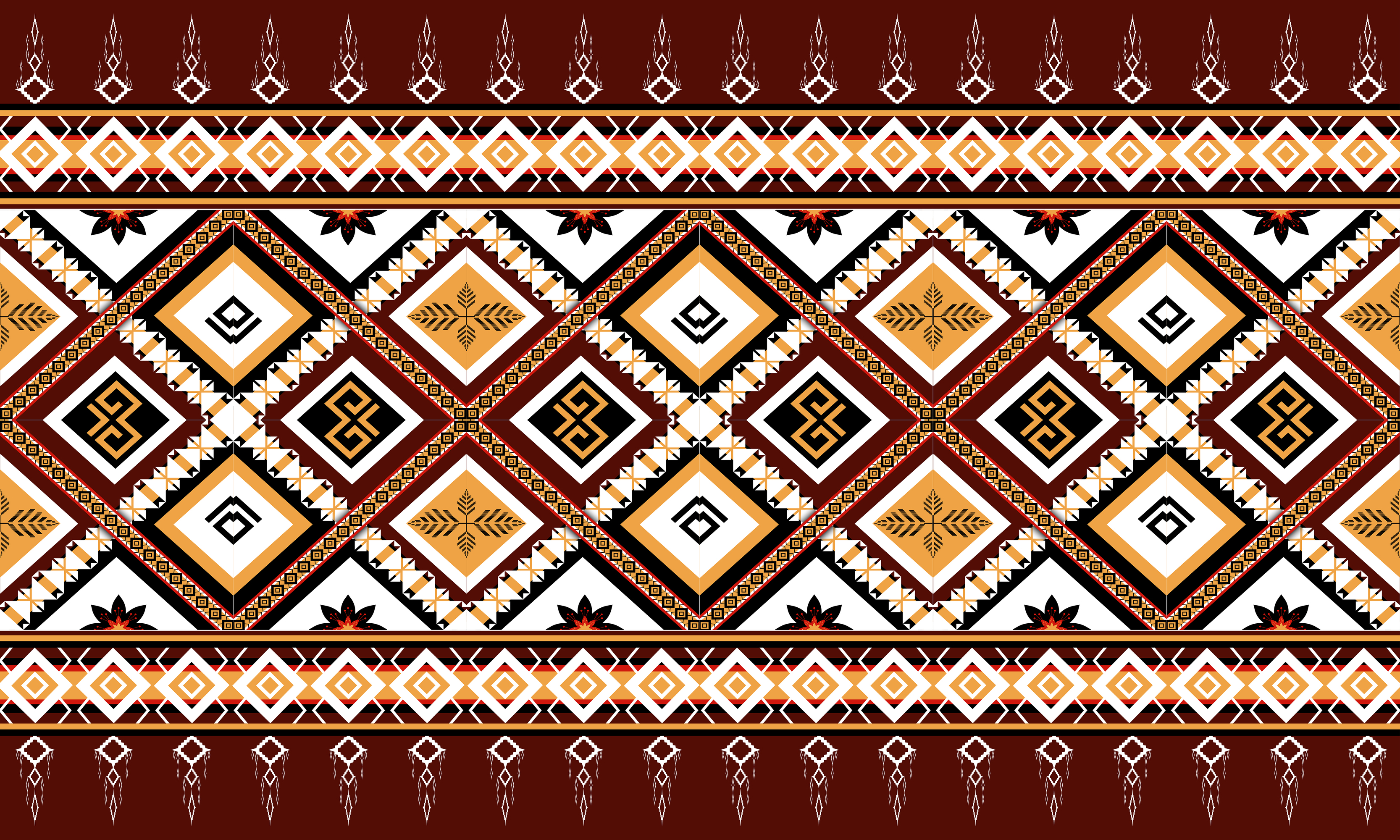The image is a richly detailed Aztec tapestry or flag, showcasing a burgundy or maroon backdrop interspersed with vibrant white, yellow, and black hues. Dominated by intricate geometric designs, the tapestry features an array of intertwined triangles and diamonds. At the image's core, there's a cross-hatched or grid pattern comprised of large diamonds, each containing four smaller diamonds. Adding to the visual complexity, triangles flank these diamonds on all sides. The top section of the tapestry transitions into a dark red zone adorned with white, square, and diamond motifs, including rows of white diamonds set against a yellow and reddish background. Below this, a yellow pathway anchors a series of large squares, each filled with unique patterns and shapes. The overall design is symmetrically mirrored on the bottom half of the image, ensuring a cohesive and harmonious visual experience.